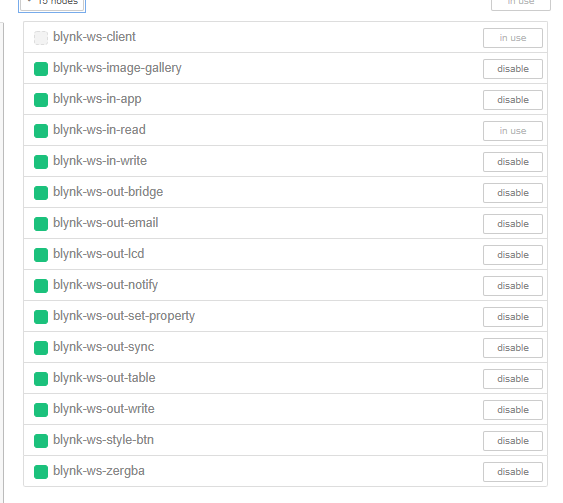The image appears to be a screenshot of a computer interface with a white background and gray text. The interface shows a list of items, each preceded by a checkbox. The list starts with an item labeled "BLYNK-WS-CLIENT," which is highlighted in gray, indicating it is selected. To the right of this label, the status "in use" is displayed. Below this, there are approximately 15 more items, each with a green-checked checkbox, indicating that they are clicked or selected. The second item in the list is labeled "BLYNK-WSIMG-GALLERY," and its status on the right side reads "disable." Most of the other items in the list also have statuses that read "disable," except for another item further down the list labeled "BLYNK-WS-IN-RED," which is also marked as "in use." This indicates that out of all the items listed, only "BLYNK-WS-CLIENT" and "BLYNK-WS-IN-RED" are active, while the rest are in a disabled state.